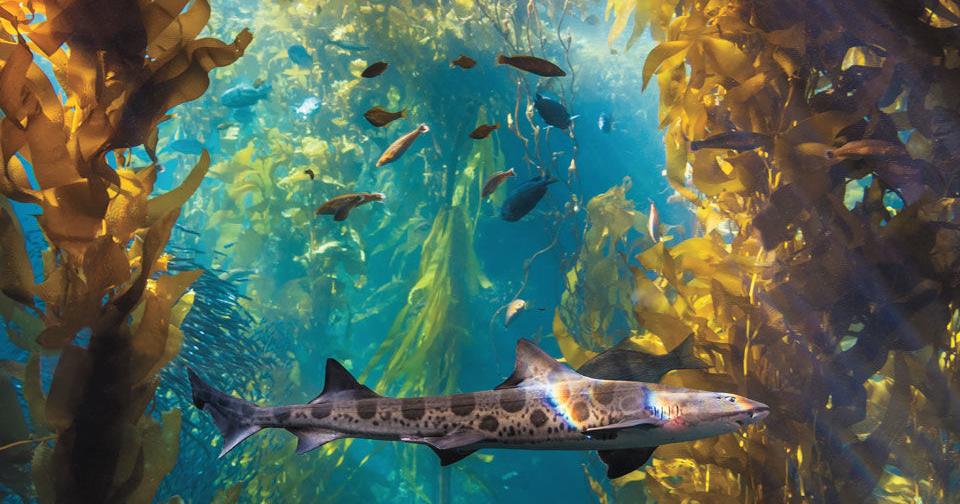A stunning, horizontally-oriented color photograph captures the enchanting underwater realm of a kelp forest. Tall, yellow seaweed frames both the left and right sides of the image, while more kelp billows upward in the background. The vibrant underwater scene is teeming with life, as schools of small fish swim gracefully throughout the water, creating an active and dynamic atmosphere. In the foreground, center stage, is a striking shark, showcasing a mesmerizing blend of colors. Its body glows with a mauve hue, complemented by distinctive brown spots scattered along its dorsal and lateral sides. The shark's pointy nose and large fins, including a pronounced dorsal fin, further accentuate its graceful, elongated form. The sunlight pierces through the water, casting ethereal rays that highlight the fish's unique markings and the overall mystical ambiance of the underwater landscape. The palette of this image incorporates an array of colors, from blue and amber to light green and dark gray, adding to the depth and richness of this vivid aquatic tableau.